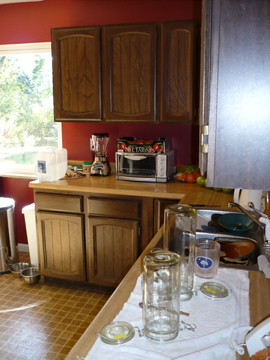This is a detailed color photograph of a cozy indoor kitchen corner. On the left side, a sizable clear window partially visible, offers a glimpse of blurry greenery outside. The far wall is painted in a rich red, contrasting with the brownish countertop below. Above and below the countertop, there are dark brown cabinets – two upper and two lower. Resting on the back countertop are a toaster oven and a blender. 

To the right, the kitchen corner continues with the countertop extending towards the viewer. A stainless steel sink is prominently featured on this section, along with a white tablecloth spread out beside it. Several clear kitchen objects are arranged neatly on the tablecloth. The edge of another dark cabinet is also visible, reflecting light possibly due to a camera flash, adding a touch of brightness to the scene.